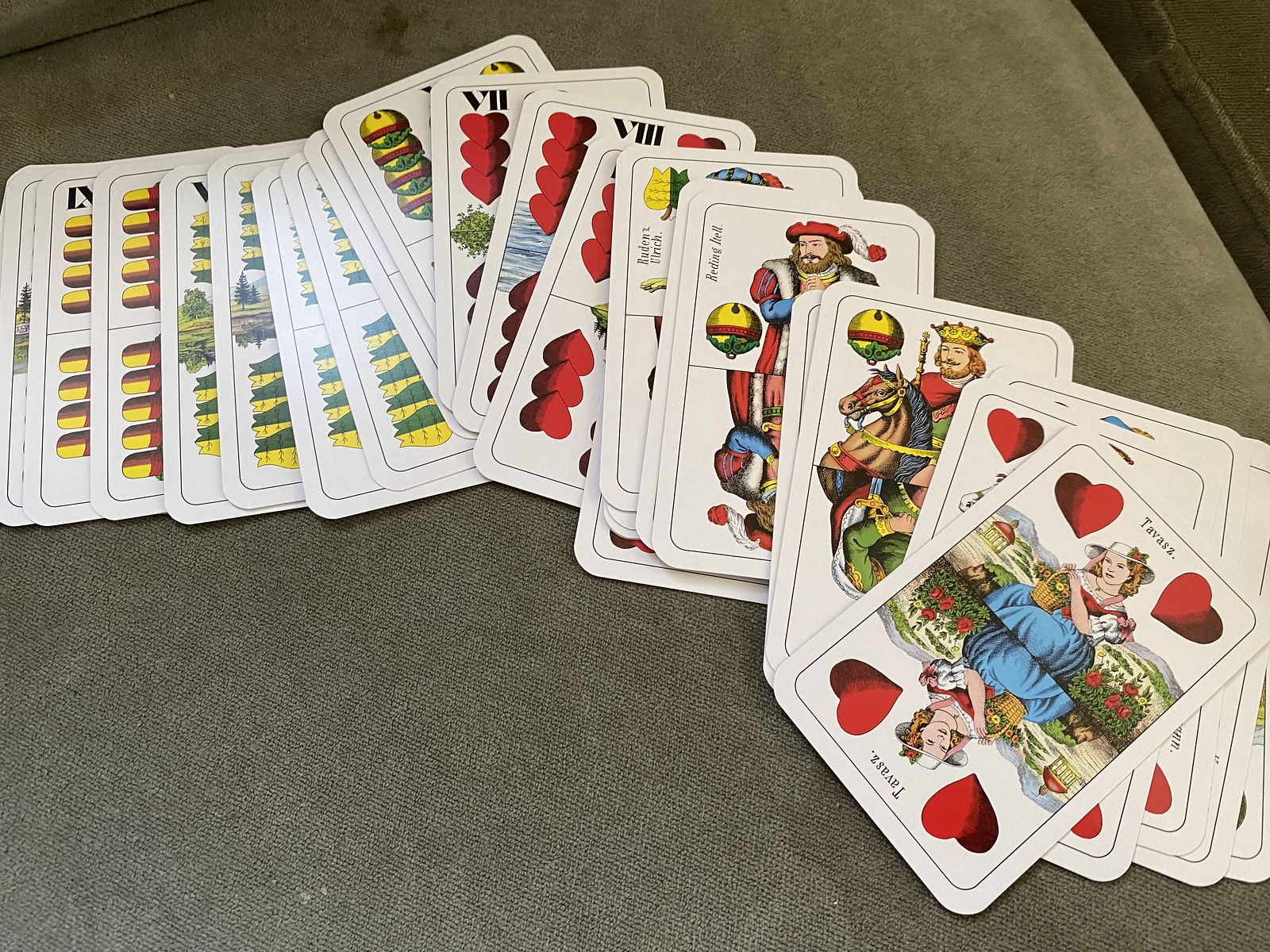A scattered set of playing cards is displayed on what appears to be a round surface, perhaps a rug or the seat of a couch. The scene includes the visible edge of a brown armrest and what looks like a black or brown magazine holder at the end of the couch. Each card in the set showcases unique and detailed illustrations. One card, the Four of Hearts, features a charming young girl adorned in a blue dress, with a red bodice and white sleeves. She sports a broad hat over her blonde hair and holds a basket amidst a quaint garden backdrop. Another card depicts a majestic king wearing a golden crown, riding a horse while donning a red robe and gripping a scepter. The lower cards in the stack reveal additional images, including a set of five shimmering gold bars and another card portraying five golden ears of corn.